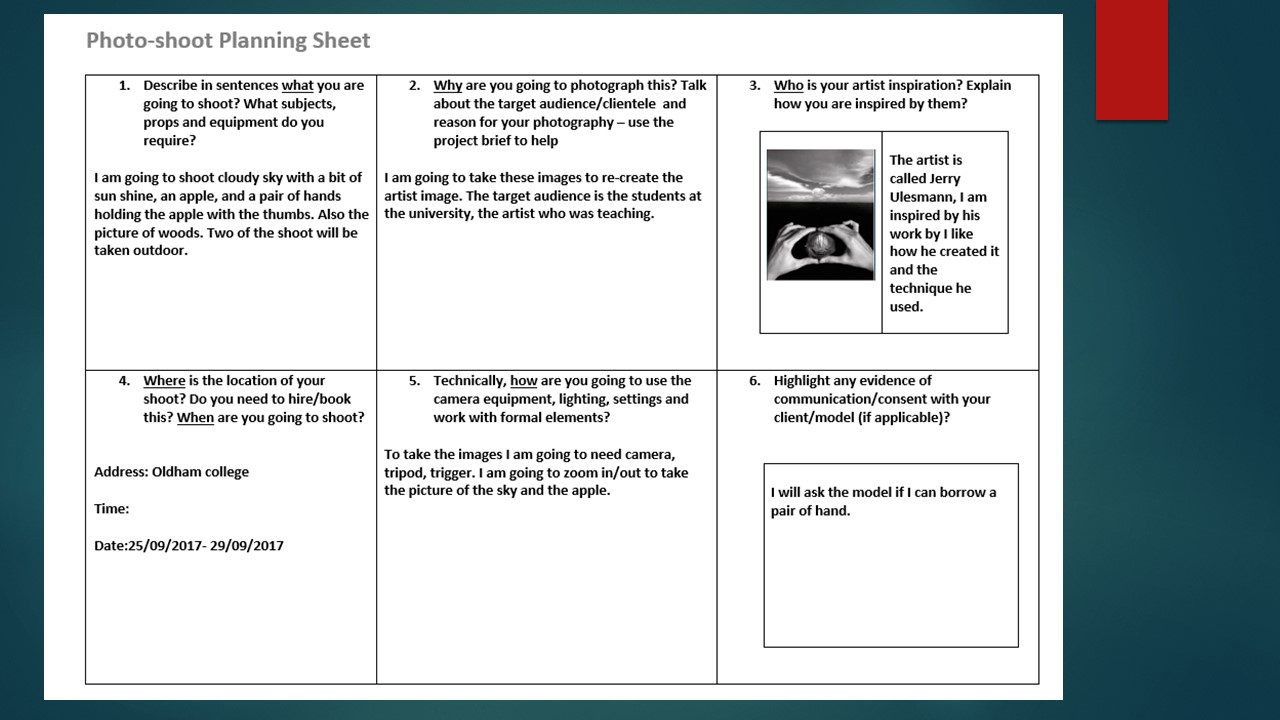This image is a detailed screenshot of a Photoshoot Planning Sheet set against a deep green background with a red rectangle in the top right corner. The sheet, which primarily occupies the white space on the picture, is divided into six numbered sections, each outlining a specific aspect of the photoshoot plan.

1. **Shoot Description**: The shoot includes capturing images of a cloudy sky with some sunshine, an apple, a pair of hands holding the apple with their thumbs visible, and a picture of woods. The shoot will primarily take place outdoors.
  
2. **Purpose and Audience**: The purpose of these photographs is to recreate an artist's image for a project targeted at university students. The inspiration comes from the artist's teachings.
  
3. **Artist Inspiration**: The artist named Jerry Uelsmann inspires this work. The photographer admires his unique techniques, especially a particular image featuring two hands holding a ball.
  
4. **Location and Timing**: The shoot is scheduled to take place at Oldham College between the 25th and 29th of September, 2017. The photographer needs to confirm the booking for this location.
  
5. **Technical Details**: The project requires specific equipment including a camera, tripod, and trigger. The photographer plans to use zoom features for close-ups of the sky and the apple.
  
6. **Communication and Consent**: The final section notes the photographer's intention to ask a model for consent to use their hands in the shoot.

Overall, this planning sheet comprehensively details the creative and logistical aspects of the intended photoshoot.